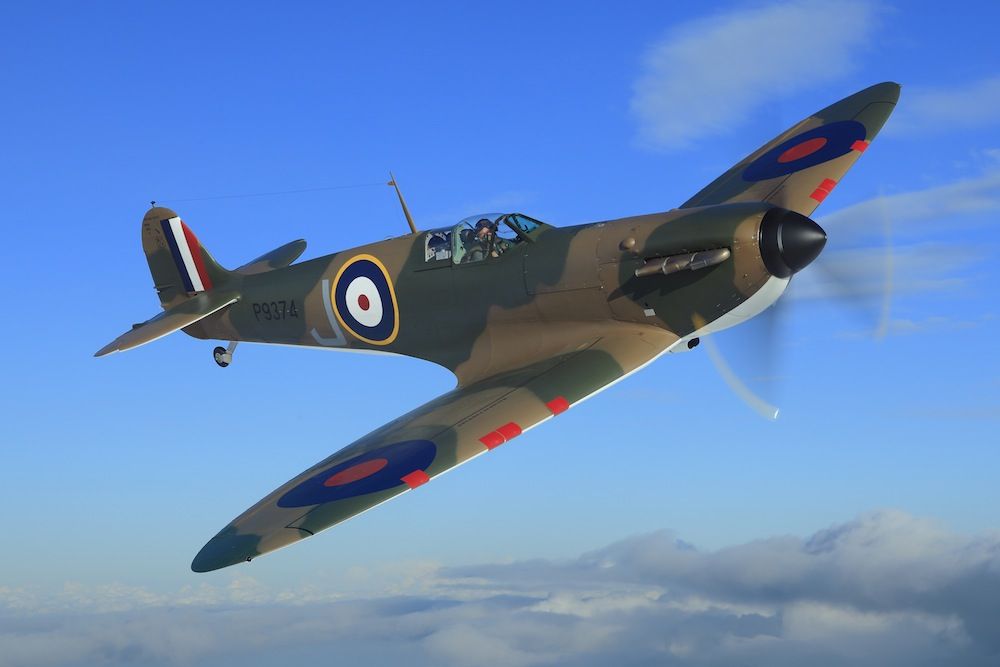The image depicts a French fighter pilot maneuvering an aircraft in mid-flight on a bright, sunny day with a few clouds scattered below. The plane, featuring a clear-topped pilot's cabin, is slightly slanted, possibly indicating a turn. The aircraft sports a dark green and light green, almost olive body with a black propeller nose. On the tail, the French flag's vertical stripes of blue, white, and red confirm its nationality. The identifier "P9374" is emblazoned in black text on the tail. The wings and the side of the aircraft showcase multiple insignias: a bullseye-like symbol with concentric circles of yellow, blue, white, and red, and additional blue circles with red centers on the wings. The pilot, the sole occupant, is visible looking down as he navigates through the mostly blue sky adorned with both thick and wispy clouds.